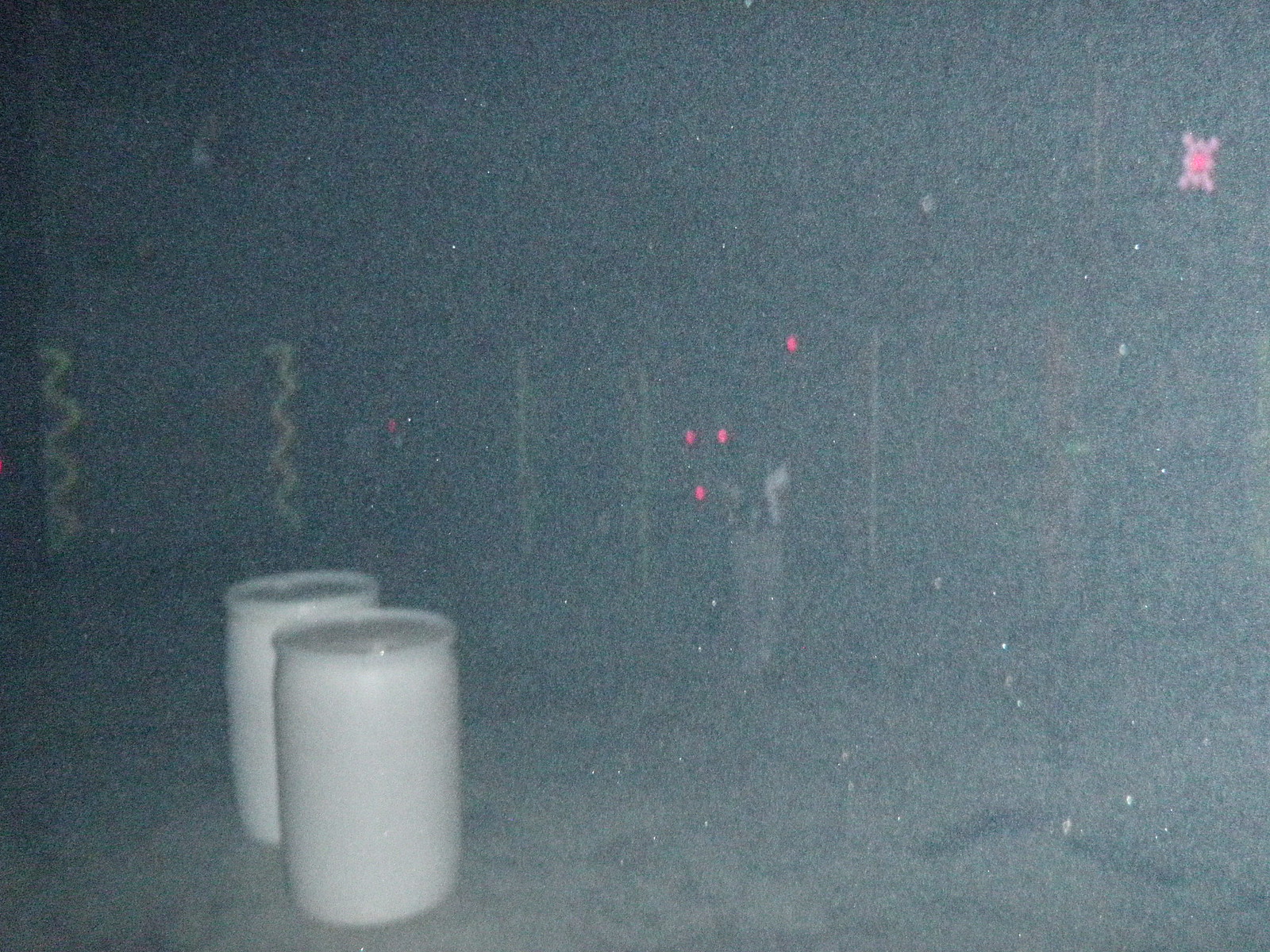This mysterious and unusual photograph, characterized by its poor quality and haziness, seems to capture a dark, possibly nighttime scene that's difficult to fully discern. Central to the image are two large, upright, white barrels with lids, positioned on the lower left side. The unusual white barrels, commonly associated with storing large items, hint at an evocative, perhaps eerie, narrative. Near the middle of the frame is a faint figure of a person wearing a black t-shirt and jeans, moving away from the camera. Above and around this figure are several small red lights, forming a triangle with one additional light to the right, creating an element of intrigue. The background is overwhelmingly dark and gray, adding to the mysterious ambiance, with some illumination coming from the lower right. To the upper right of the photograph, a distinctive pink circle with lines resembling spikes and a bright pink dot in its center, paired with various dark and wavy lines, adds to the enigmatic vibe. This detailed blend of disjointed elements and unclear visuals forms a genuinely perplexing and atmospheric image.